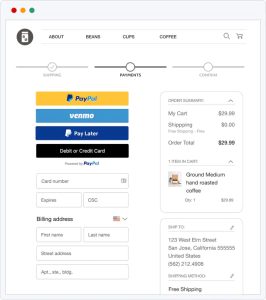In the upper left corner of the image, there are three small horizontal dots in red, yellow, and green. Below these dots is a gray circle. To the right of this circle, in gray text, are the labels "Adjust," "Cups," and "Coffee." Directly beneath these labels is a long gray line with a circle at its center.

Below this section, several payment options are displayed, each within color-coded boxes: "PayPal" in yellow, "Venmo" in blue, "Pay Later" in dark blue, and "Debit or Credit Card" in black. 

Further down, there are empty text fields with faint placeholder text for "Card Number," "First Name," "Last Name," and "Street Address," all grouped under the heading "Billing Address."

To the right of these fields, the "Order Total" is prominently displayed as $23.98 in dark text. Below this, the product description reads "Ground Medium Hand-Roasted Coffee" in black text. The shipping address and phone number are located in the lower right corner, accompanied by "Free Shipping" in black text.

In the upper right corner, beside the word "Coffee," there is an image of a magnifying glass and a shopping cart icon.